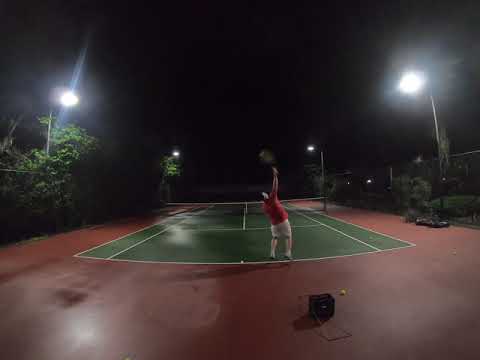The square image, taken at night, features a black sky devoid of any lights or sun. The scene is a bit blurry but clearly depicts an outdoor tennis court. The court's edges are tannish red, with the playing surface itself being green marked by white lines. On each side of the court, in the upper left and upper right corners, there are blurred streetlights casting a dim glow over the scene. Centered in the image is a man playing tennis, appearing to be in the midst of serving. His right arm is stretched upwards, holding a black tennis racket with yellow netting. He wears a red short-sleeved shirt, white shorts, and white shoes. The court is flanked by trees and enclosed by a wire fence. Two black pillars support a white and black net stretched across the court. On the ground to the man's left lies a yellow tennis ball, with another further toward the foreground near a small black box, possibly a ball hopper.